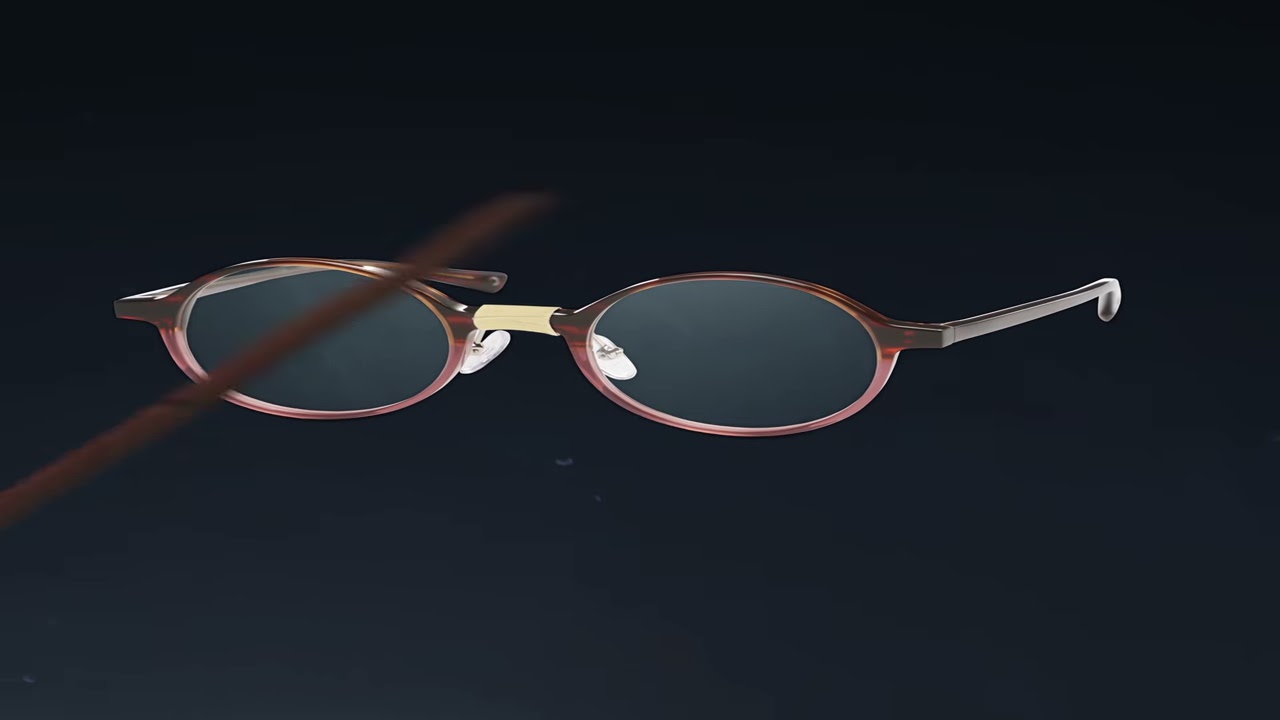The image features a pair of glasses with oval-shaped lenses, framed by a thin, brownish-red frame that displays noticeable striations. The coloration of the frame darkens progressively towards the earpieces. At the center of the glasses, a cream-colored, tape-like strip connects the lenses and is supplemented by a light beige nose piece with visible nose rests. The background is predominantly dark, varying from black to dark grey and blue shades, with faint light seeming to filter through the lenses. Protruding from the left side of the image is a fuzzy, out-of-focus stick-like object, which appears brown and stretches diagonally across the glasses.